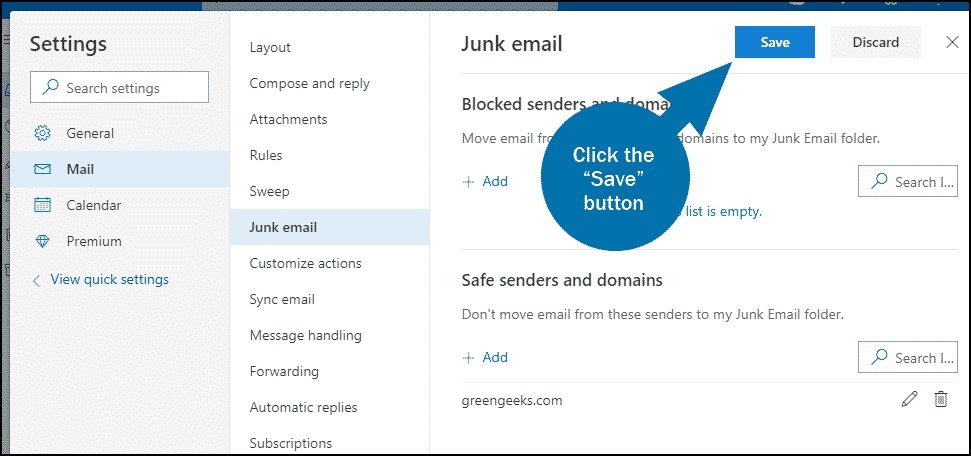This image depicts a settings pop-up window with a detailed configuration layout. On the left-hand side, there is a vertical menu labeled "Top Settings" at the top. Below this label, the menu items are arranged sequentially: "Upload Settings," followed by a "Search Settings" bar, "General," "Mail," "Calendar," and finally "Premium." At the bottom of this vertical menu, there is an option labeled "View Quick Settings" accompanied by a left-pointing back arrow.

In the center section, we observe the "Mail" options menu, which has been selected, revealing its specific settings. On the far right side of the window, there's an additional vertical submenu within the "Mail" settings. Here, the "Junk Email" option is selected, opening a detailed view of the junk email settings.

In this detailed view on the right, the header "Junk Email" is prominently displayed on the upper left-hand side. Below this header, there is a blue circular icon with an arrow pointing to the right. This icon is labeled "Save" and is clearly pointing to a blue "Save" button, emphasizing the action needed to save the junk email settings.

Overall, the image captures an intricate settings interface with multiple levels of menus, clearly labeled and organized, with a specific focus on configuring junk email settings.